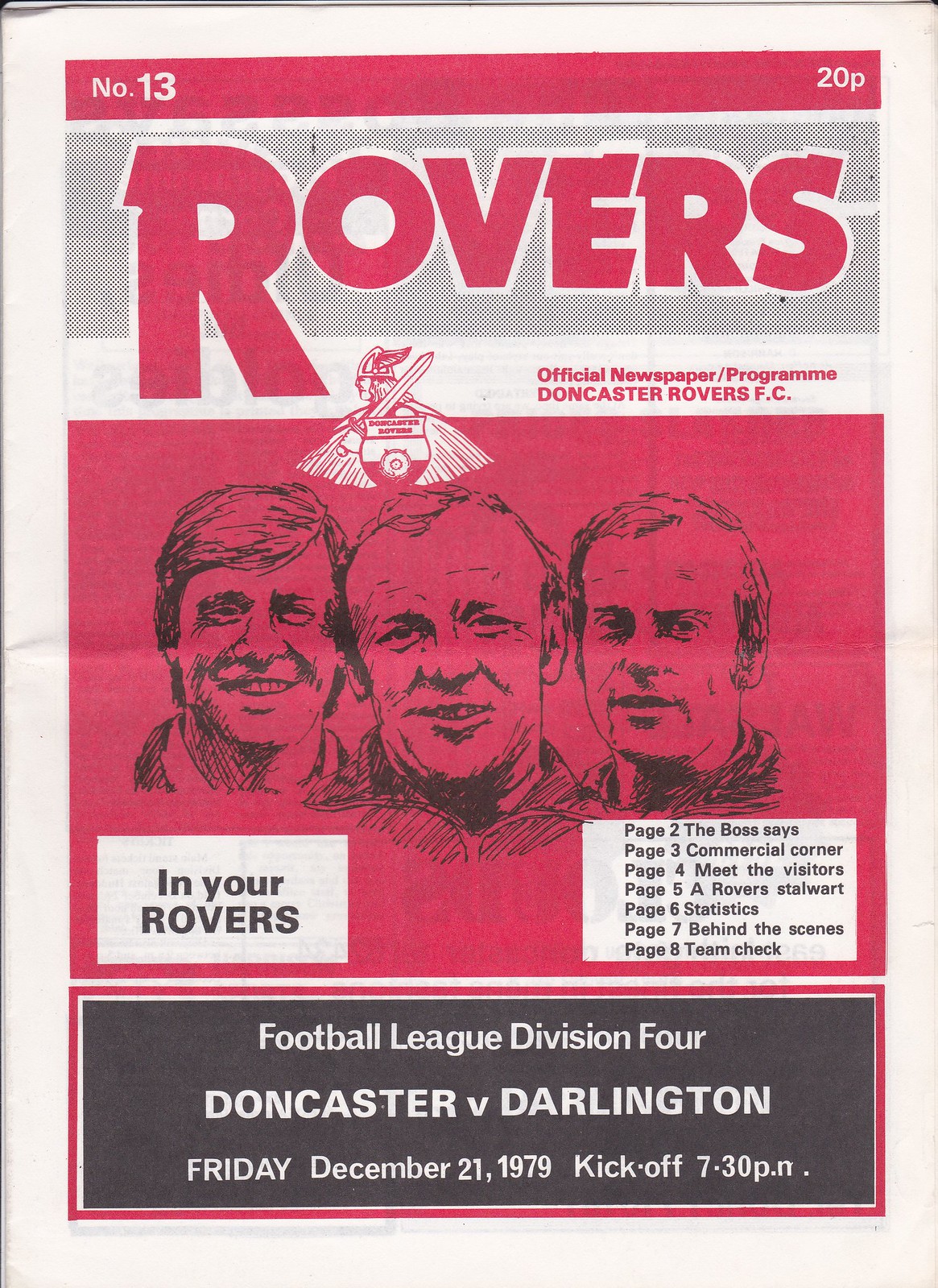This image showcases a color photograph of a vintage red and black printed program cover for "Rovers." Dominating the top is the title "ROVERS" in bold red letters against a gray rectangular background, with an enlarged "R" leading the title. Above this title is a red bar stretching horizontally, indicating "Number 13" on the left and "20P" on the right. Below the main title, a large red rectangle features black sketches of three men's faces side by side, giving the appearance of a drawing. Positioned to the left of this illustration is a white box with black text that reads, "In Your Rovers."

To the right of the portraits, page guides list contents from Page 2 through Page 8, detailing sections such as "Page 2: The Boss Says," "Page 3: Commercial Corner," "Page 4: Meet the Visitors," "Page 5: A Rover Stalwart," "Page 6: Statistics," "Page 7: Behind the Scenes," and "Page 8: Team Check." At the bottom of the cover, a black rectangle prominently displays the match information in white text: "Football League Division 4, Doncaster versus Darlington, Friday, December 21st, 1979, kickoff 7:30 p.m." The entire design exudes the style of a vintage publication print, evoking nostalgia for a past era of football programs.